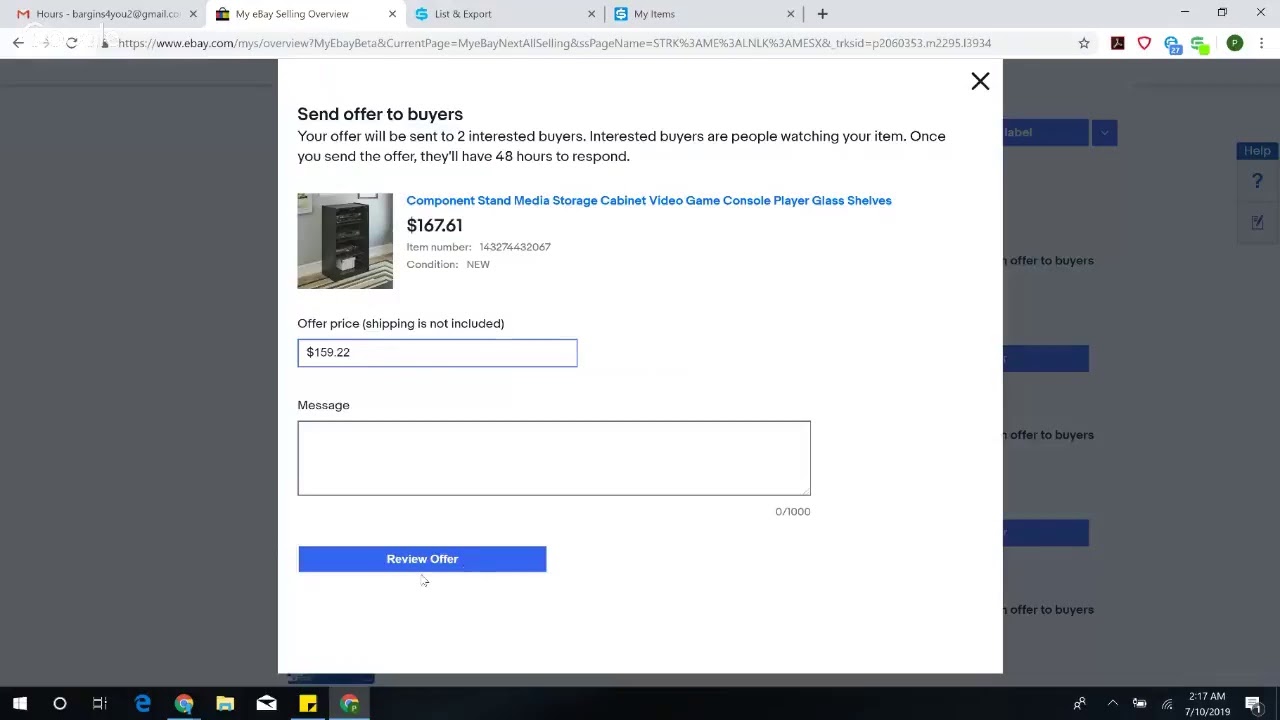This image is a screenshot of a computer screen displaying a web browser with multiple open tabs and a pop-up window overlaid on an eBay listing page. At the top of the screen, there are four open browser tabs: the first tab shows the Gmail logo with its distinctive white and red envelope icon, followed by a tab labeled "eBay" that features a multicolored shopping bag icon in black, blue, yellow, and red. The third tab is titled "List and Export," displaying a blue icon, and the fourth tab, partially unreadable, features a blurred blue icon.

The browser window includes control icons such as a gray plus sign, a minus sign, a window resize icon, and a red X for closing the browser. Below this, the address bar contains navigation buttons—a back arrow, a forward arrow, and a refresh icon—along with a star for bookmarking, a black square, a red shield, and several icons in blue, green, and green with a white letter. To the far right, three vertical black dots indicate additional browser settings.

The main content of the screen displays the eBay website. The background of the site is grayed out, accented with blue boxes and black text. A white pop-up box titled "Send Offer to Buyers" is prominently featured in the center. The box has a black X in the top right corner for closing the message. It states, "Your offer will be sent to two interested buyers. Interested buyers are people watching your item. Once you send the offer, they will have 48 hours to respond" in black text.

Within the pop-up, details of a product listing are provided. A blue header reads "Component Stand, Media Storage, Cabinet, Video Game, Console Player, Glass Shelves," accompanied by an image of a black media storage unit against a gray wall with a visible floor. The listing indicates the price as $167.61 and notes the item condition as new. There is a section for entering an offer price, with a pre-filled value of $159.22 in a box next to the note "shipping is not included." Below this, there is an empty message box and a blue button labeled "Review Offer" in white text.

The bottom of the screen features a black taskbar with several icons: a Windows logo, a white circle, a white speaker symbol, a blue 'E' for Internet Explorer, two Chrome icons, a manila folder icon, an envelope icon, a yellow box, some character icons in white, an upward arrow, a battery icon, a Wi-Fi symbol, and a digital clock displaying the date and time from the year 2019, albeit a bit blurry.